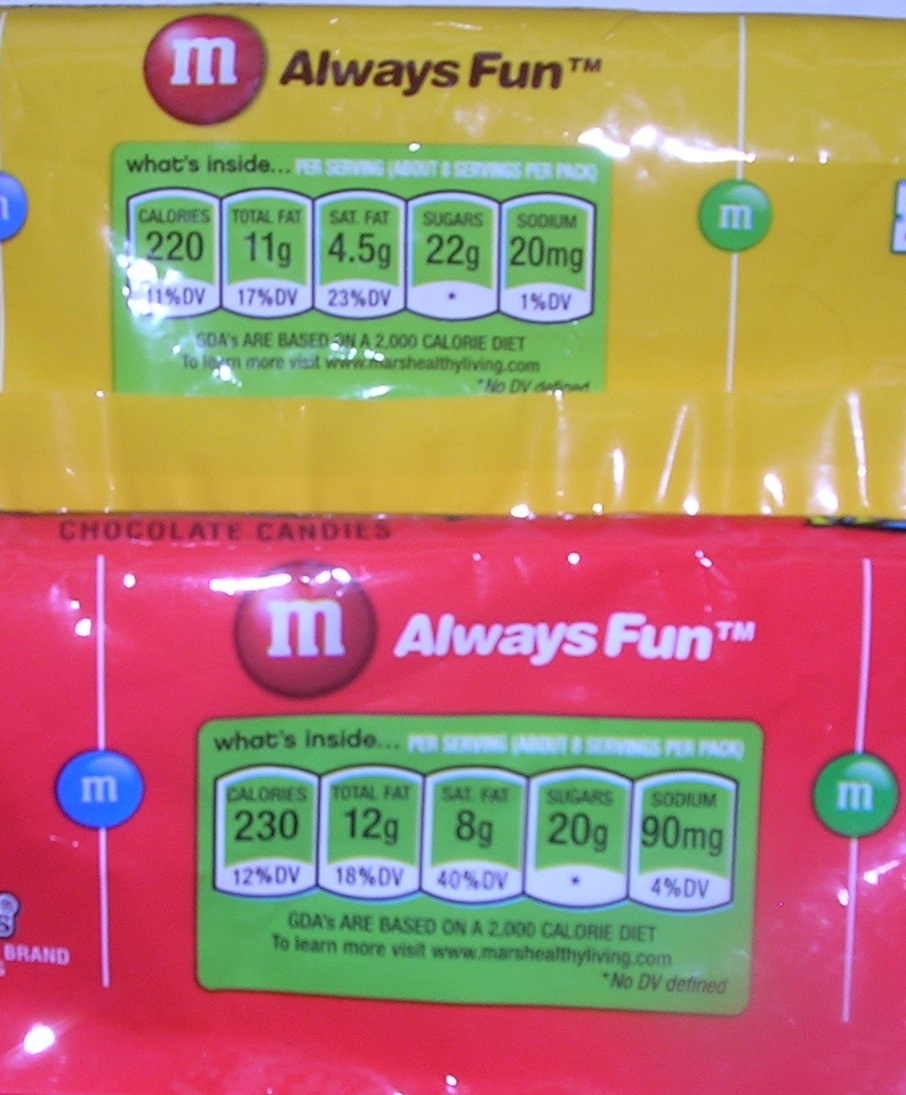The image depicts the back of two M&M's candy packages, highlighting their nutritional information. The top package is yellow, likely representing Peanut M&M's, and features a green nutrition label. The label indicates that a serving size has 220 calories, 11 grams of total fat, 4.5 grams of saturated fat, 22 grams of sugar, and 20 milligrams of sodium, with about eight servings per pack. The bottom package is a red bag of traditional M&M's, also with a green nutrition label, showing 230 calories, 12 grams of total fat, 8 grams of saturated fat, 20 grams of sugar, and 90 milligrams of sodium per serving. Both packages are adorned with images of the candies and the slogan "Always Fun." Nutritional guidelines suggest these values are based on a 2,000 calorie diet, with more details available at marshealthyliving.com.